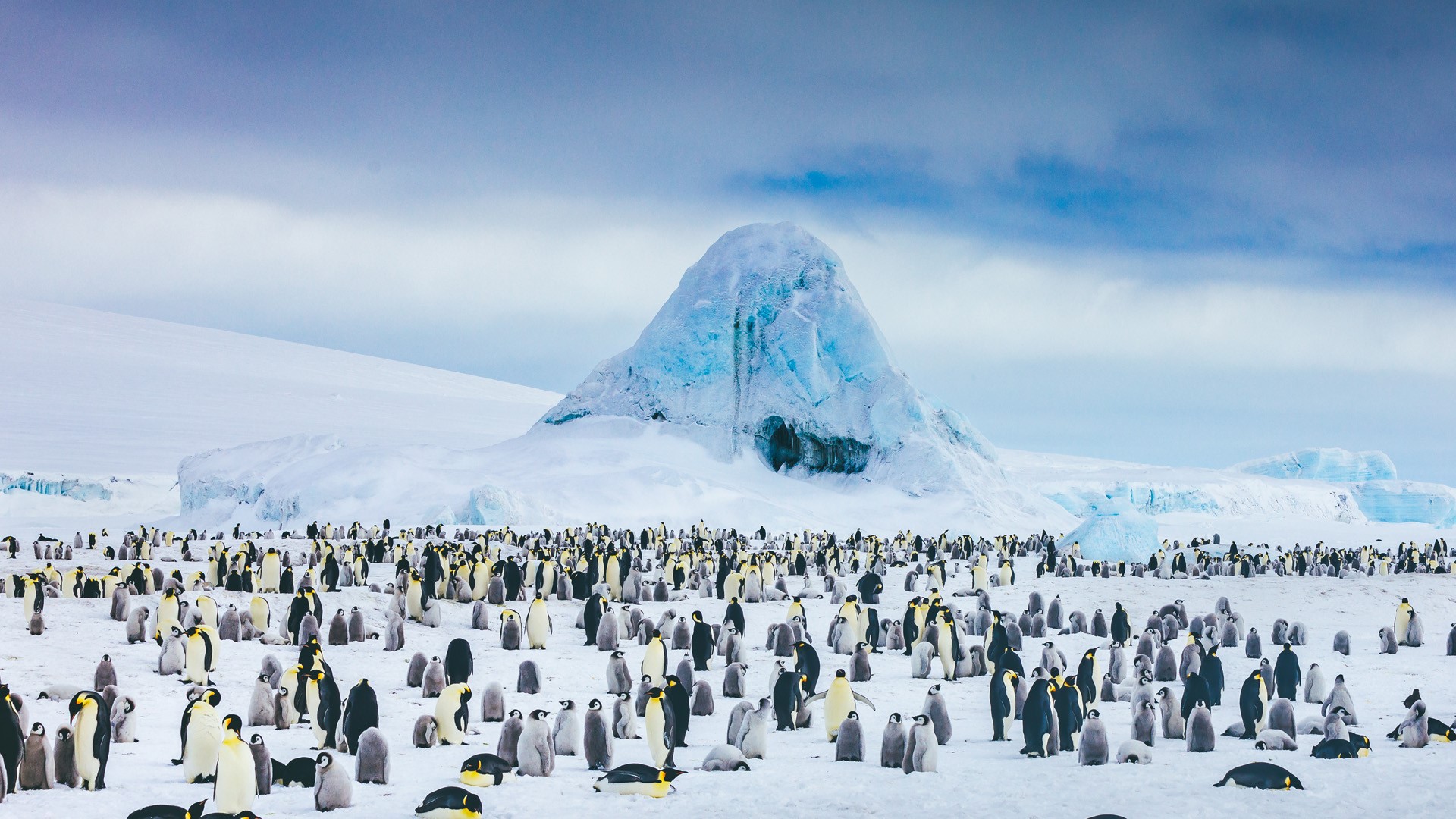The image portrays a surreal, possibly art-printed scene set in an Antarctic-like environment, where a massive congregation of hundreds, if not thousands, of penguins dominates the icy foreground. These penguins, mostly standing with a few resting or interacting in pairs, showcase their natural gray, black, and white plumage, with sporadic streaks of yellow adding a touch of color to the scene. The ground beneath them is a pristine, flat expanse of snow. In the backdrop, a strikingly triangular, sharply inclined hill or mountain, pale blue at its nucleus and enveloped in white, pierces the sky. This icy peak, seemingly either arising from the snow or emerging through wispy white clouds, adds an almost surreal touch to the composition. The deep to medium blue sky above is adorned with feathery white clouds, enhancing the otherworldly atmosphere. This captivating artwork, with its blend of realistic and fantastical elements, depicts a vibrant and dynamic natural tableau, punctuated by the intriguing icy formation at its center.